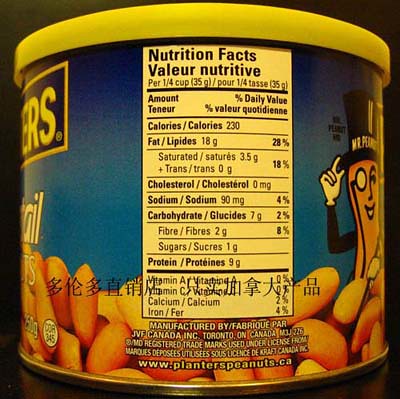The image features a cylindrical can of Planters nuts adorned with a vibrant blue label and a distinct yellow plastic cap. The iconic Mr. Peanut mascot, depicted with his monocle, top hat, and white-gloved hand holding the top hat, is prominently displayed on the right side of the can. Beneath Mr. Peanut, at the bottom of the can, are illustrations of peanuts. The label contains bilingual nutritional facts, in both English and another Asian language, specifying details such as 230 calories, 18 grams of fat, 3.5 grams of saturated fat, 0 cholesterol, 90 milligrams of sodium, 7 grams of carbohydrates, 2 grams of fiber, 1 gram of sugars, 9 grams of protein, 0 percent vitamins A and C, 2 percent calcium, and 4 percent iron. The product weight of 250 grams is noted on the left side of the can. Additional text includes the manufacturer’s details, indicating it is produced by FARC, PAR, or a similar entity and is linked to a Canadian website, planterspeanuts.ca.